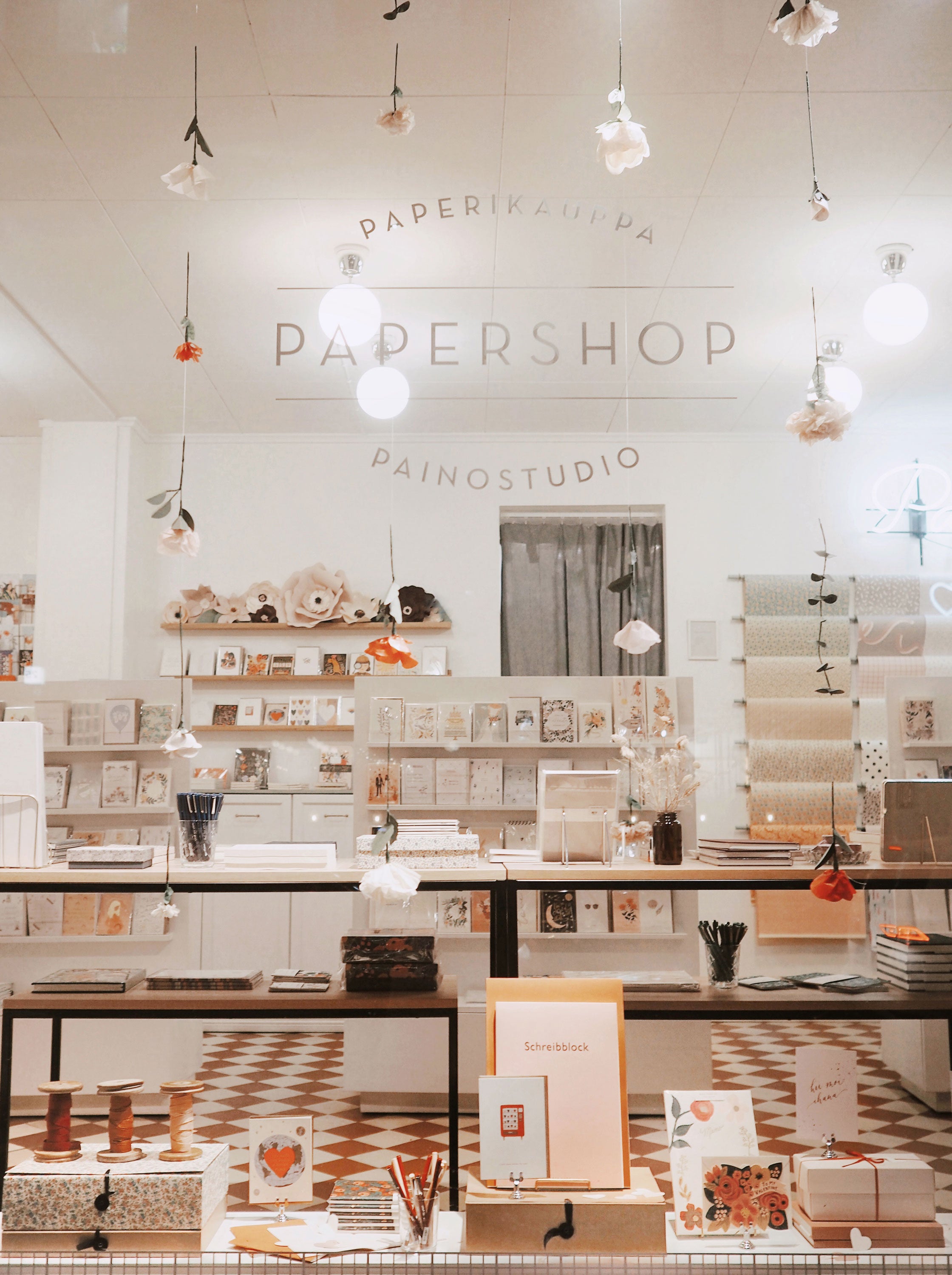The interior of the paper shop, "Pano Studio," is immaculately staged in a neat and symmetrical manner. The walls and ceiling lamps are painted white, creating a clean and bright atmosphere. Suspended from the ceiling are artificial flowers and modern round light bulbs, adding a whimsical touch to the otherwise pristine setting. The shop's floor features a distinctive checkerboard pattern in an orangish-brown and white tile. 

The shelves are lined with a variety of paper goods, including greeting cards for various occasions, small books, and paper spools in colors like light blue, pink, and light orange, reminiscent of wrapping paper. Large paper flowers and flower sculptures are artistically displayed, enhancing the store's decorative theme. Tables within the shop showcase cards, stationery, and scrapbooking papers. The counter, where customers complete their purchases, is adorned with pens, books, a bottle with flowers, and additional paper goods. 

In the background, racks and shelves hold more paper items, including greeting cards and other stationery. A separate room, indicated by a curtain, is partially visible, suggesting more space within the shop. The overall ambiance is one of meticulous organization and aesthetic charm, making "Pano Studio" a visually appealing paper shop.